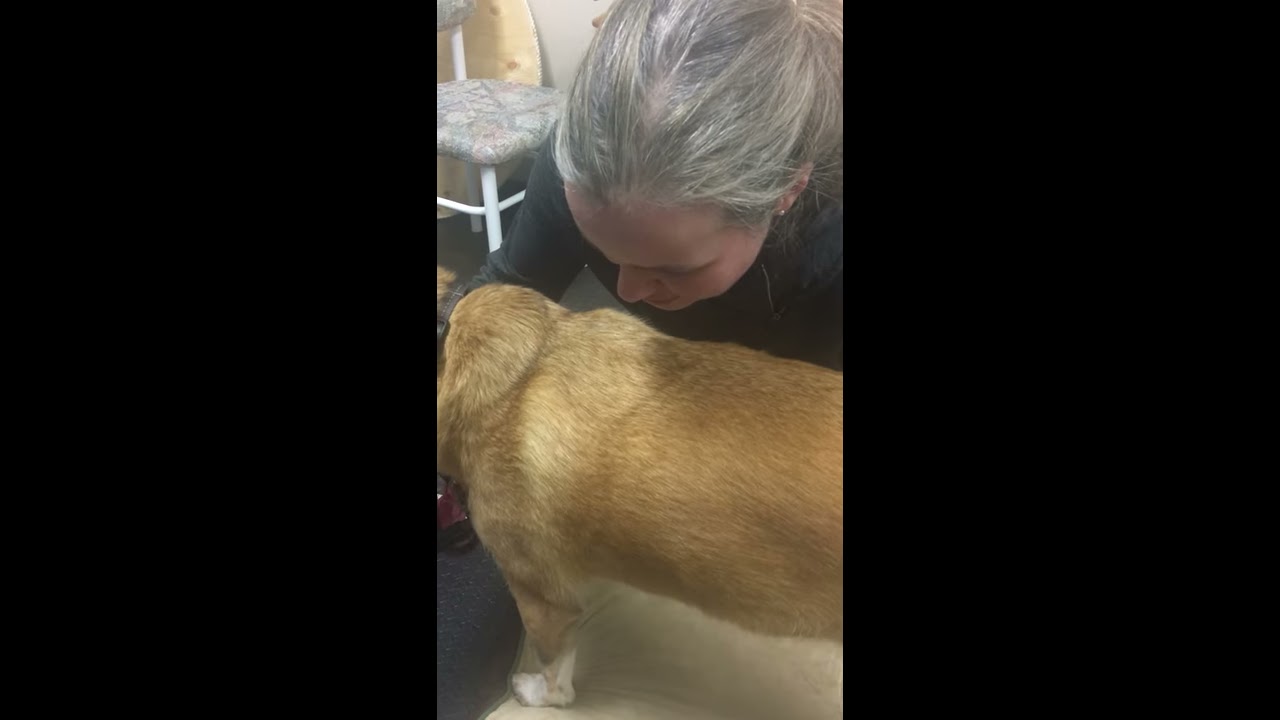The image features a close-up, portrait-oriented shot centered on an older white woman interacting with a dog. The woman, identifiable by her light skin and gray hair pulled back, is wearing a long-sleeve black shirt and small beaded earrings. She is bending over the dog, which has a long, light blonde to tawny brown coat with white paws, though its head and hindquarters are not visible. Her face is close to the dog's back, suggesting a moment of care or attention. On the left side of the background, there is a white-legged chair with a floral or gray seat cushion, set against a beige wall. Additionally, a round piece of wood or some curved object leans against the wall in the upper left corner. The large black rectangular areas on the left and right sides of the image frame the central scene, drawing focus to the woman and the dog.